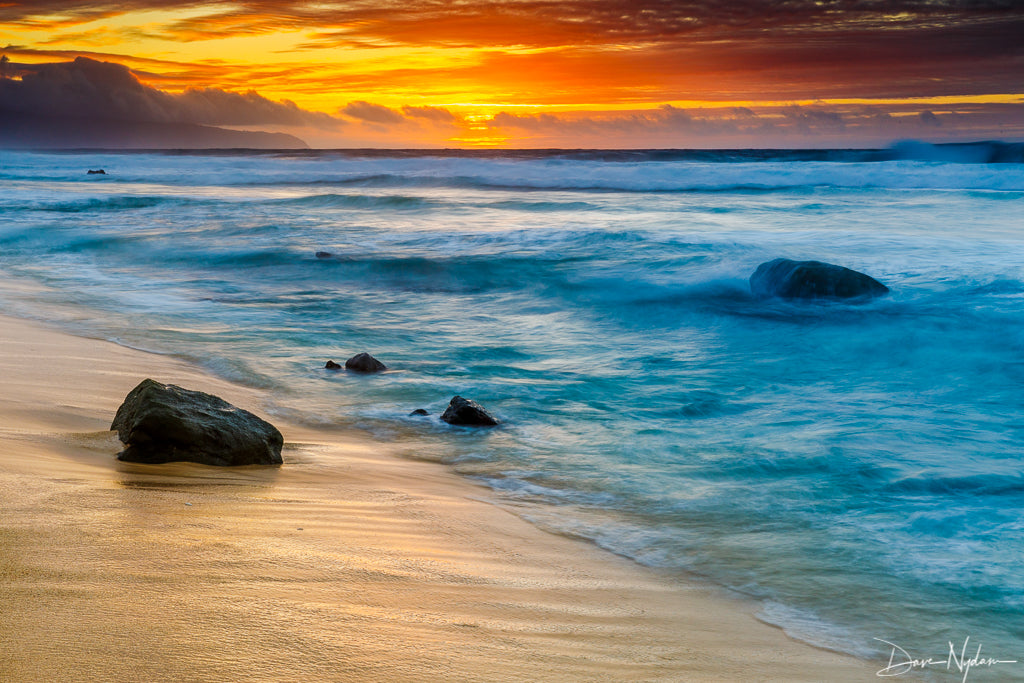The image is a vibrant painting of a beach at sunset, capturing the stunning beauty of nature with remarkable lifelike detail. The beach features beige sand and turquoise to teal blue waters, interspersed with white bubbles formed by crashing waves. Large, dark reddish-black rocks are scattered both on the sand and within the water. The sky is awash with a brilliant yellow hue, heavily tinged with orange and red, indicative of a glorious setting sun. Clouds hang overhead, adding texture to the sky. In the distance, a small ship is faintly visible. The painting is signed in white letters in the bottom right corner by the artist, possibly reading “Dan Napoleon.”